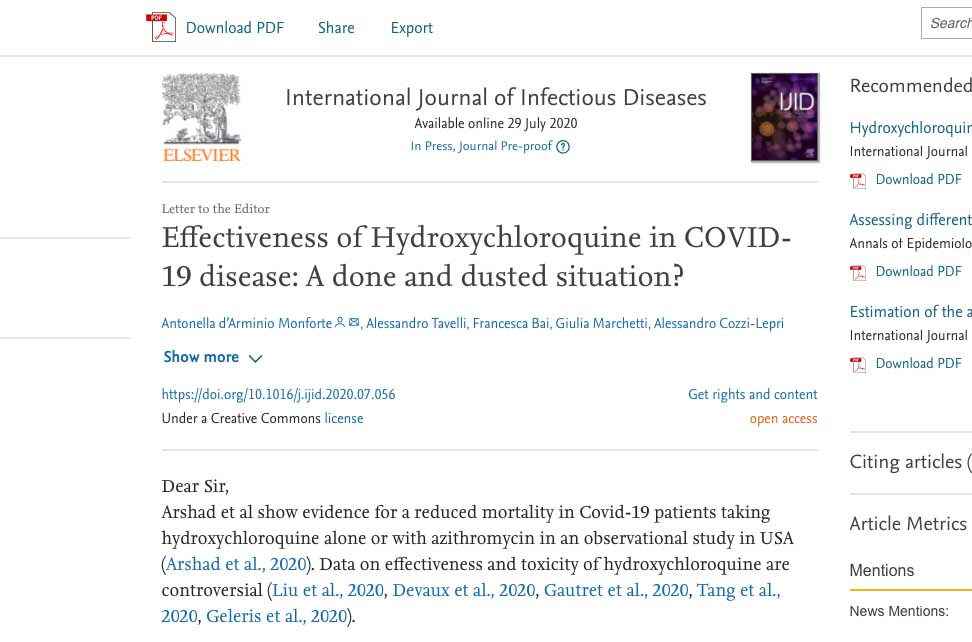**Detailed Caption:**

This image is a screenshot of a desktop version of a scholarly website, filled with a considerable amount of text and various interactive elements. In the upper left corner, there is an Acrobat PDF icon accompanied by the text "Download PDF." To the right of this icon, there are options labeled "Share" and "Export." On the far right, partially obscured by the screen edge, is a button or text box labeled "Search."

Below this top navigation line, on the left side, there is an icon depicting a tree. Beneath the tree icon, the name "Elsevier" is displayed in orange font, suggesting the logo of the renowned academic publishing company. Adjacent to this, the title "International Journal of Infectious Disease" is prominently visible, indicating either the name of the journal or an advertisement. Further detailing states "Available online 29 July 2020" in blue font, followed by a status note "In press journal pre-proof" with an accompanying question mark tooltip.

To the right of these texts, there is an abstract image with purple tones and some illegible lettering. Below this visual element, the text "Letter to the Editor" appears in small font, followed by a larger and bolded title: "Effectiveness of Hydroxychloroquine in COVID-19 Disease: A Done and Dusted Situation." 

Beneath the title, a list of author names is provided, featuring Italian surnames such as Anatella, DiRomino, and Montefiore, indicating a collaborative scholarly work. Below the authors, there is a "Show more" option alongside a URL link to order a Creative Commons license.

A snippet of the letter is also present, beginning with a salutation "Dear Sir," and mentioning a study by Arshad et al, which presents evidence of reduced mortality in COVID-19 patients treated with hydroxychloroquine alone or with azithromycin. The snippet continues to discuss controversial data regarding the effectiveness and toxicity of hydroxychloroquine, followed by references and citations.